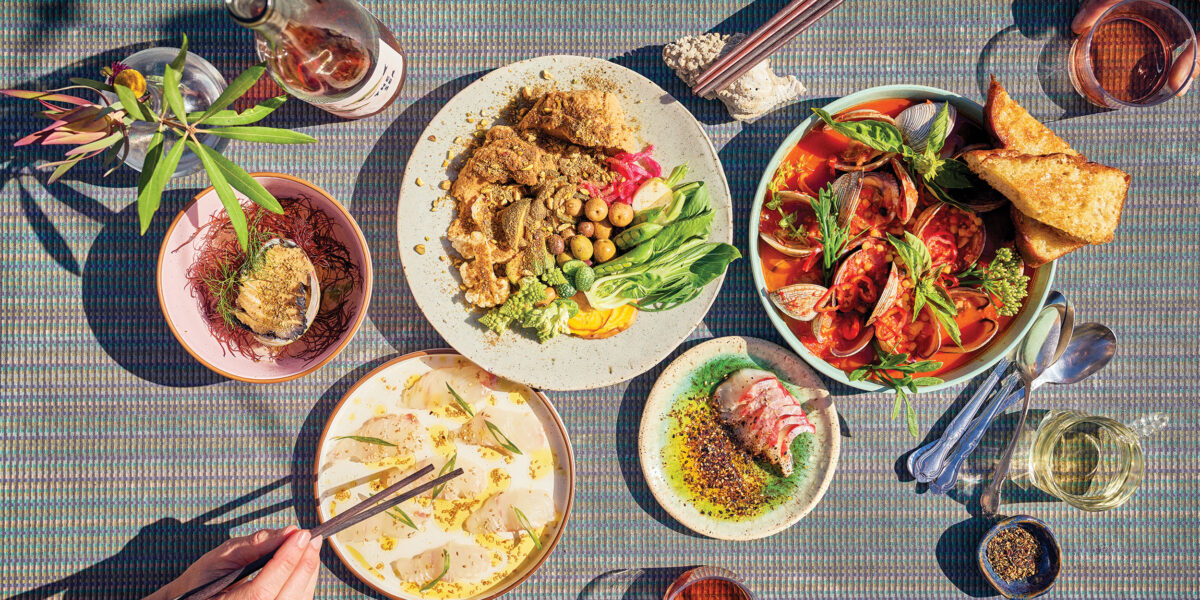This vibrant and detailed overhead photograph captures a diverse and sumptuous meal spread across a woven tablecloth adorned with gray, blue, and red lines. The table is filled with five distinct dishes, each presented in separate bowls or plates. 

In the lower left, a hand is seen entering the frame, skillfully wielding chopsticks to pick up beige-colored dumplings garnished with finely chopped green onions from a round plate. To the right of the dumplings, a smaller round plate hosts succulent, cut-up ribs adorned with green garnishes underneath them.

Adjacent to the ribs, an elegant array of silverware, including three spoons, can be observed alongside a small bowl containing ground pepper. Centered on the table, a large dish holds a medley of roasted chicken, olives, onions, and squash, displaying a colorful and hearty vegetable spread. 

Further to the right, a larger bowl contains clams or oysters nestled in a red sauce, topped with green garnishes, and flanked by two pieces of toast resting on the side of the bowl. A sophisticated touch is added by the presence of a smaller bowl containing what appears to be a deviled egg, meticulously garnished.

A bottle of red liquid, possibly wine, and various drinking glasses, including one with an olive, add to the luxurious ambiance of the table setting. Scattered throughout are additional elements such as bread, tomatoes, lettuce, and an assortment of nuts and vegetables, contributing to the vivid palette of brown, red, green, black, gray, and yellow hues. The overall impression is one of an elaborate and fancy meal, likely prepared with great care and attention to detail.